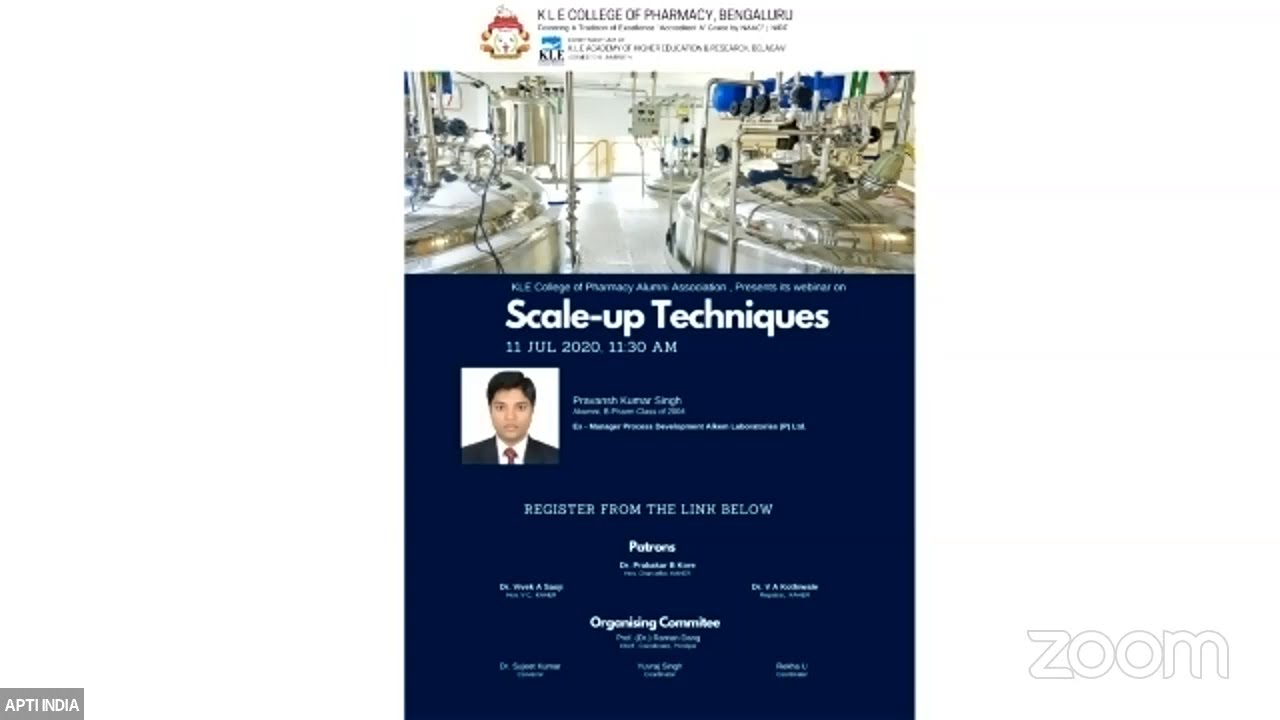The image depicts a webpage section, likely a contact or informational section, featuring a prominently placed poster centered on a white background. The poster has a navy blue background with "Scale Up Techniques" in large white letters at the top, along with the date "11 July 2020" and the time "11:30 a.m." Below these headers is a photograph of a laboratory with two large metal tanks in a white metal room, suggesting a brewery or similar facility. The poster also includes a professional headshot of a middle-aged man in a suit and red tie on the left side. Adjacent to his image are details about a class or seminar, indicating participation information and registration details. The bottom-left corner of the poster mentions "APTI India," and the bottom-right corner is marked with the "Zoom" logo, indicating the event's platform. Additionally, the poster highlights the "KLE College of Pharmacy" and provides links for registration, emphasizing an educational event organized by the institution.